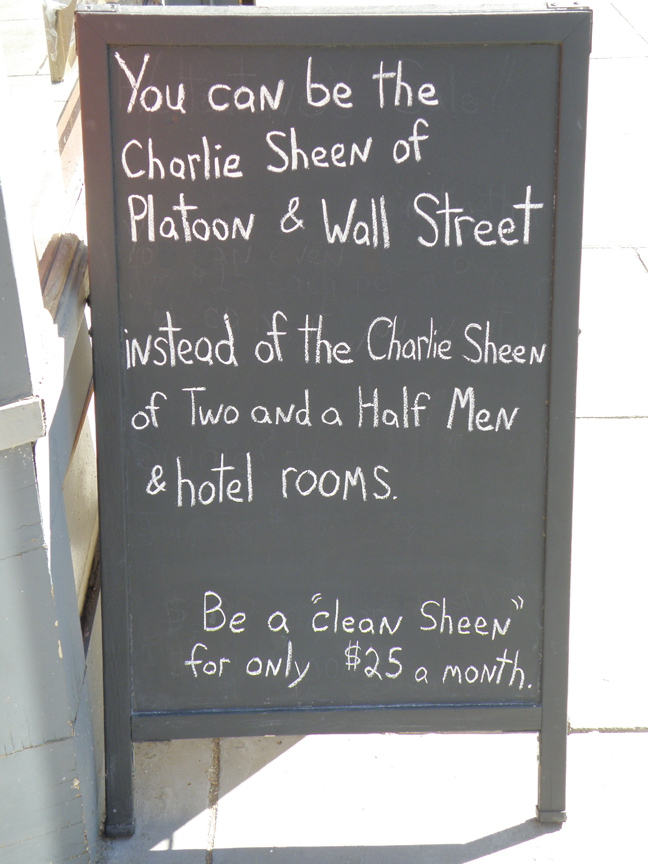The image depicts an outdoor advertisement featuring a black A-frame chalkboard standing upright on a concrete sidewalk, bathed in daylight with visible shadows. The chalkboard, situated next to a stone building, displays a message in white chalk lettering. The text reads: "You can be the Charlie Sheen of Platoon on Wall Street instead of the Charlie Sheen of Two and a Half Men and Hotel Rooms. Be a 'clean Sheen' for only $25 a month." The board, primarily in black and white, hints at a promotional offer, possibly for a self-improvement or lifestyle service.